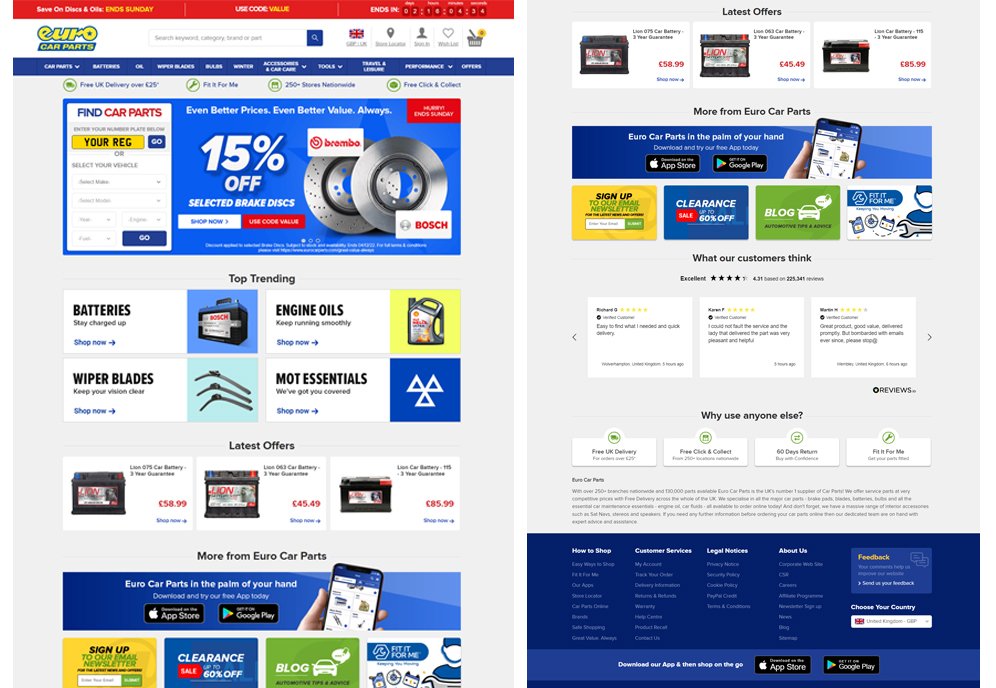This image displays a detailed digital catalog for a car parts store.

**Left Page:**
- **Header Area:**
  - **Design:** A vibrant red band stretches across the top.
  - **Background:** Subtle grey.
  - **Title:** “Euro Car Parts” banner.
    - **Font Details:** 
      - “Euro” in elegant, blue-outlined lowercase cursive.
      - “Car Parts” in bold yellow uppercase letters, set on a blue background.

- **Navigation and Functions:**
  - **Search Bar and Icons:** Options for changing country, selecting location, logging in, liking items, and accessing the shopping cart.

- **Main Content:**
  - **Promotions:**
    - Large blue box announcing “15% off selected brake discs” with a visual of brake discs.
  - **Clickable Sections:**
    - Quick access buttons for various categories such as batteries, engine oils, wiper blades, and MOT essentials.
  - **Additional Products:** Various items listed underneath these sections.

**Right Page:**
- **Content Highlights:**
  - Top portion displaying various batteries.
  - A link to download the store’s app from the App Store or Google Play.
  - Newsletter sign-up option.

- **Customer Interaction:**
  - Section showcasing customer reviews.

- **Footer:**
  - Standard informational links including customer service details, legal notices, and information about the company.

This well-organized catalog efficiently presents the store’s offerings, promotional deals, and user-friendly navigation for automotive enthusiasts and shoppers.